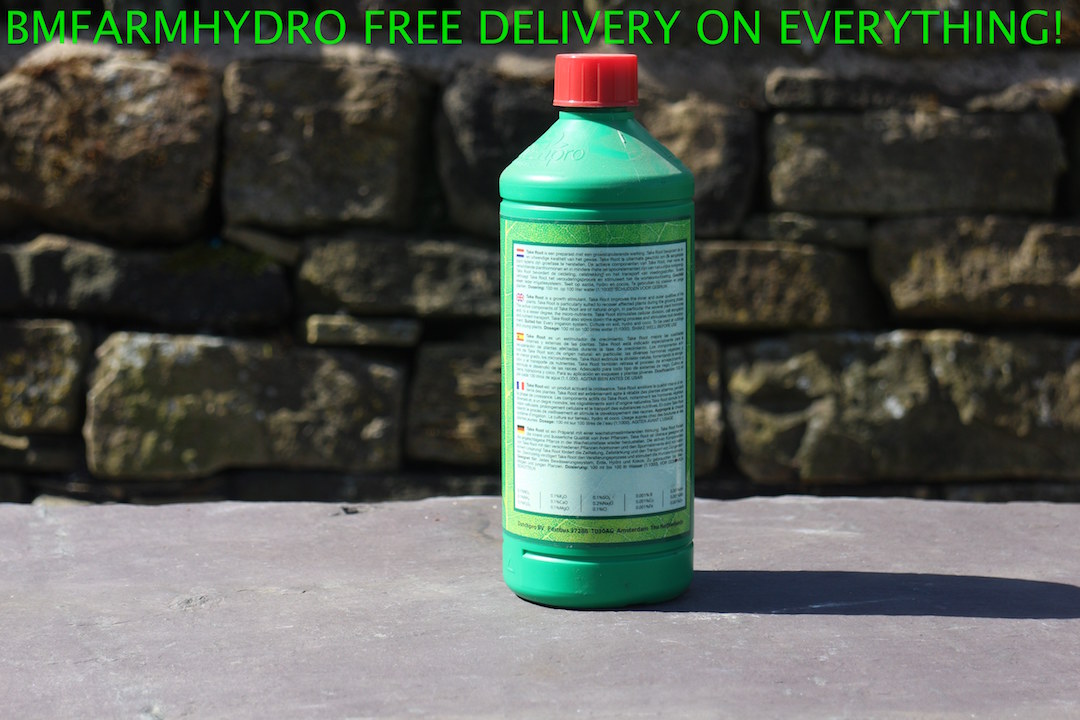In this image, a central green bottle with a red lid and a prominent white label adorned with roughly five paragraphs of text and a light green border stands out on a stone surface. Positioned outdoors in the middle of the day, the setting exudes a casual yet natural ambiance. The background showcases a stone brick wall composed of three distinct rows of stones, each with a mix of gray, brown, white, and black hues. The stones occupy slightly more than half of the picture's height, while the stone ground beneath the bottle fills the remainder. At the top of the image, bold text reads "BM Farm Hydro, free delivery on everything!", emphasizing the advertisement style of the scene.